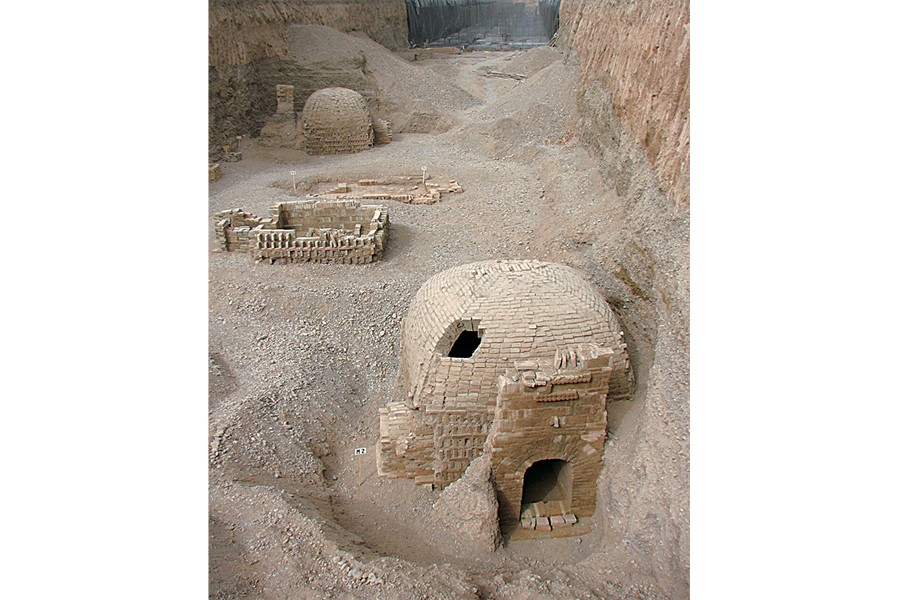The image depicts an archaeological excavation site revealing the remnants of an ancient city, set against tall, rugged rock cliffs on either side. In the foreground, a partially unearthed main structure stands prominently, characterized by its tan-colored bricks and a dome with a small hole at the top. The entryway is arched and transitions into a rectangular form, and nearby, there's evidence of a balcony with railings. Surrounding the structure is a landscape laden with piles of stone and gravel, with dirt and earth deliberately excavated around it. Behind the main structure, a smaller, squarish building with an open, damaged roof can be seen, along with another domed building in the distance. The background features a distinctive black wall, appearing almost burnt, with a gravel path leading down from it. The entire scene captures the essence of an archaeological dig, revealing ancient architectural elements and a primitive-style home carved out from the surrounding landscape.